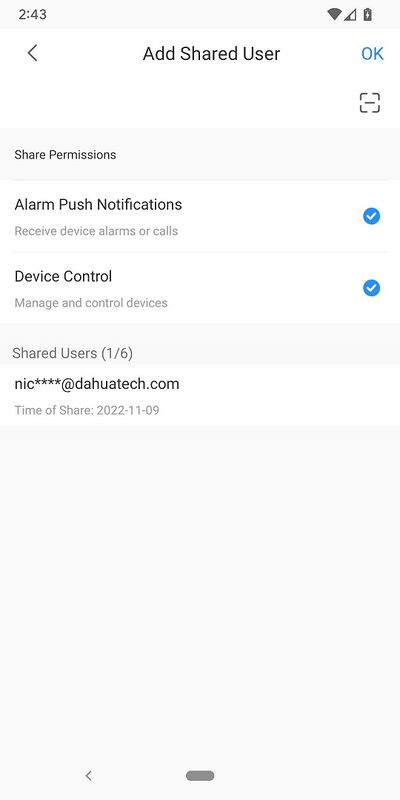The screenshot displayed in a vertically rectangular frame captures a moment from a cell phone screen. At the top, the time "2:43" is positioned on a thin light gray horizontal bar alongside Wi-Fi signal and battery icons located to the far right. Below this, on a white background centered text reads "Add Shared User." On the left side of this interface, a back arrow is shown while a blue "Okay" button is positioned on the right.

Below this section, a gray horizontal banner reads "Share Permissions." Further down, on a white background, two items are listed: "Alarm Push Notifications," which notes that the user can receive device alarms or calls, and "Device Control," indicating the user can manage and control devices. Both options are marked with a white check mark inside a blue circle.

Continuing downward, on a light gray background, it indicates "Shared users 1 of 6," followed by an obscured email address formatted as "****@bahuatech.com." The timestamp for this share action is "2022-11-9."